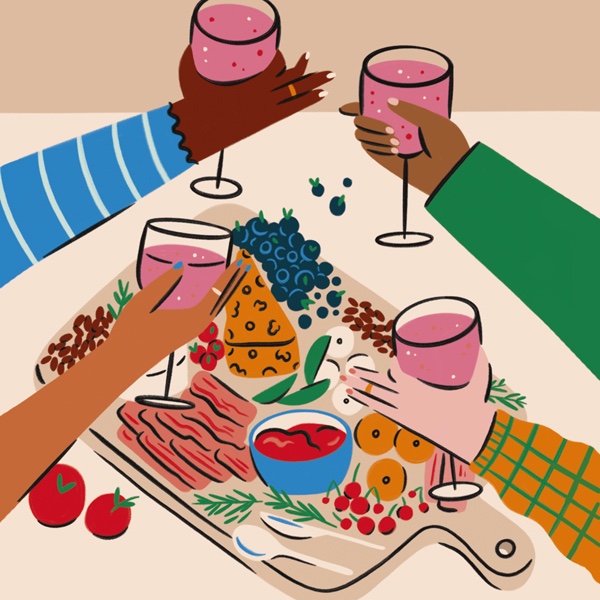This vivid computer-animated illustration captures a festive moment of four diverse hands holding wine glasses in a toast over a table laden with an abundant spread. The image is stark with no shading, using bold blocks of color. There are four distinct hands reaching in from the edges of the square frame, each sporting different sleeves: a black hand in a white and blue striped shirt with painted fingernails and a ring, a brown hand with blue nail polish, a white hand in a yellow and green checkered sleeve, and another black hand in a green sleeve. Each hand raises a glass filled with a pinkish liquid. Below, on the beige table, lies a cutting board crowded with various food items including cheeses, meats, tomatoes, grapes, cherries, blueberries, oranges, and a bowl of an unidentified red substance. This image encapsulates a moment of shared celebration, richly detailed in both culinary and cultural diversity.